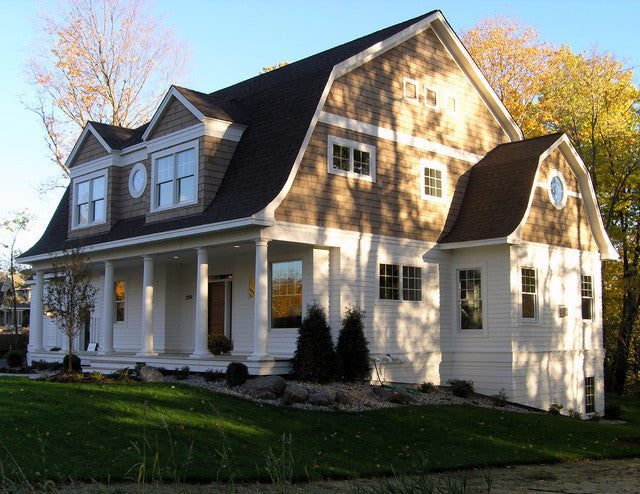This image captures a stunning and expansive Dutch colonial house bathed in the light of a bright, sunny day. The house stands prominently with its elegant design featuring wooden white siding on the bottom half and brown cedar shakes on the upper portion, all trimmed in white. A large, dark gray shingled roof extends down to a grand front porch supported by five imposing columns, creating a robust and inviting entrance. The house, appearing to be three stories high with added dormer windows, is surrounded by a lush, meticulously manicured lawn that is rich and dark green.

In front of the house, a smaller tree and additional plantings accentuate the vivid greenery. On either side of the house, larger trees with bright green foliage contribute to the picturesque setting, though one tree in the background displays yellow leaves, hinting at the transition into fall. Serene blue skies stretch overhead, while dappled sunlight casts gentle beams on the right side of the house and the verdant treetops, highlighting the harmonious blend of natural and man-made beauty. The surrounding landscaping includes scattered rock formations, adding to the overall aesthetic charm.